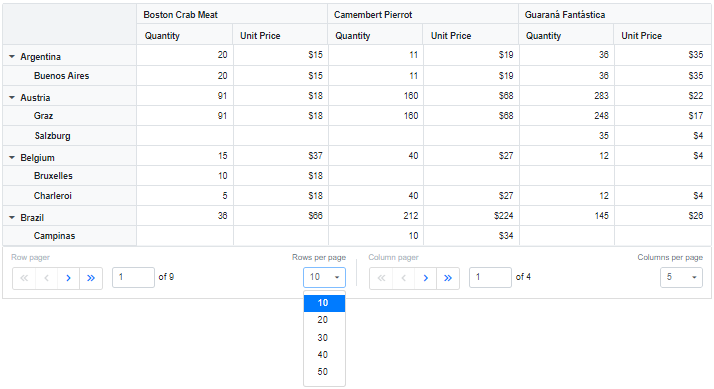This image depicts a comprehensive data chart titled "Boston Crab Meat." It features three main sections: the first for "Boston Crab Meat," the second for "Camarade Period," and the third for "Granada Fantastica," each with dedicated columns for quantity and unit price.

On the left side, the chart lists several countries along with specific cities for each. For Argentina, the city listed is Buenos Aires. Austria includes Graz and Salzburg, Belgium lists Brussels and Charleroi, and Brazil shows Campinas.

The chart offers various filters and pagination options. It indicates that this is page 1 of 9, with rows per page set to 10, adjustable to increments of 20, 30, 40, or 50. Additionally, there is a column pager indicating that it is on page 1 of 4, with the columns per page currently set to 5.

Visually, most of the text is rendered in black, while the columns are shaded grey against a white background, enhancing readability. This detailed layout effectively organizes and presents extensive data in an accessible format.